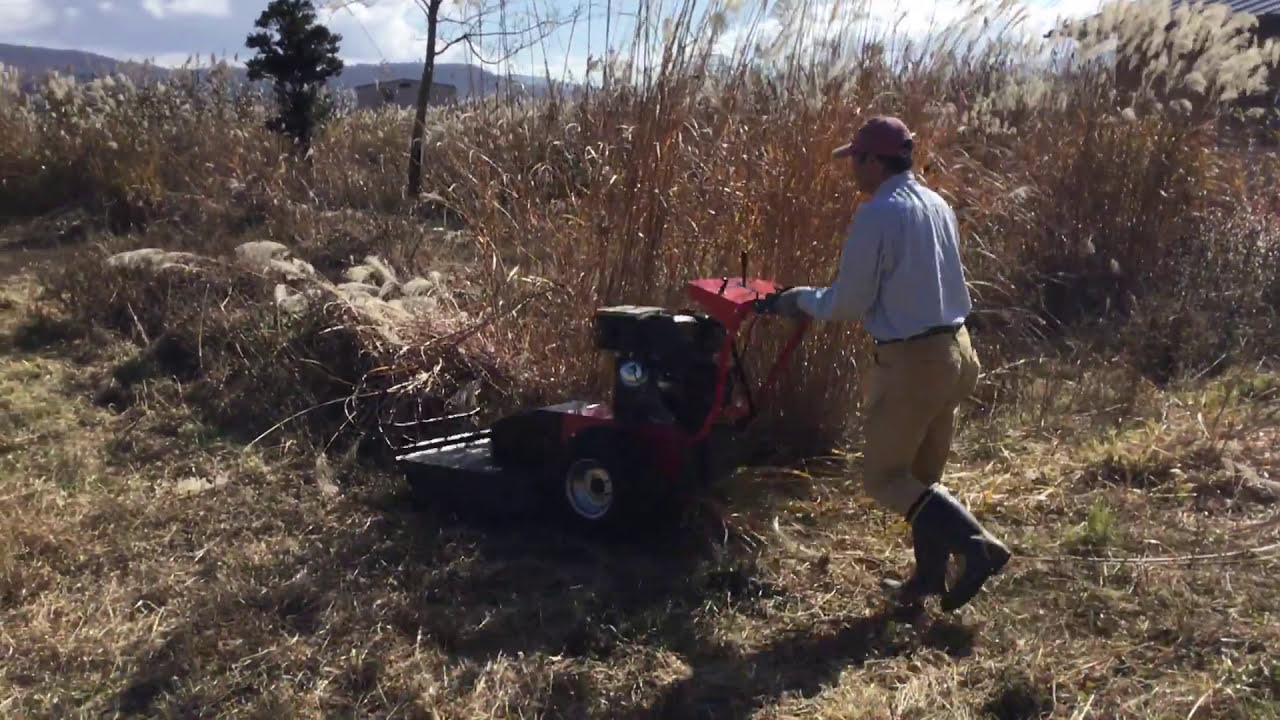In this detailed outdoor photograph, a man with a dark skin tone is seen mowing a very tall, dry, beige grass, resembling pampas grass, using a red push lawn mower or harvester. Positioned centrally in the image, he is viewed mostly from the side and back, facing slightly to the left. He wears a long-sleeve blue shirt, khaki pants, black rain boots, and a purple baseball cap. The overgrown field he is working in stretches out into the distance, with more thick brush visible throughout. The sky above is light blue with some scattered clouds. In the background to the upper left, there are green trees, a little house, and the outline of distant mountains, giving a sense of the expansive outdoor setting. The scene, bathed in daylight, emphasizes the man's effort in taming the hay-like grass amidst a natural, rustic landscape.